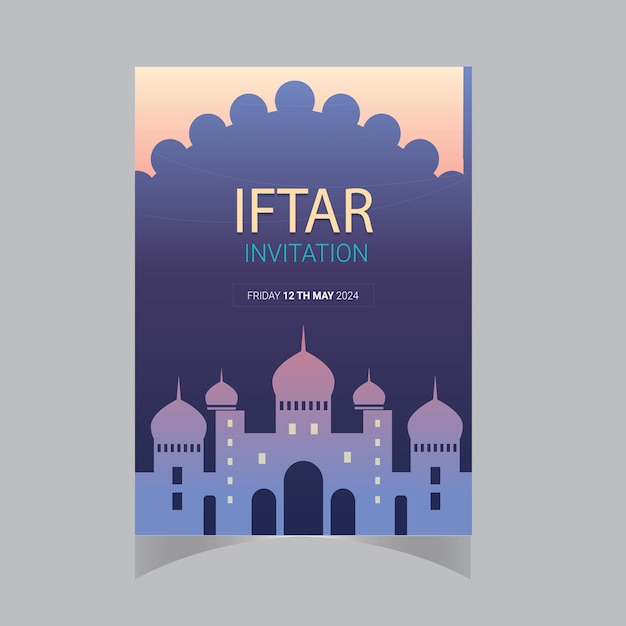The image depicts a beautifully designed invitation card for an Iftar event, scheduled for Friday, 12th May 2024. The card features text in the center stating "Iftar Invitation" in capitalized letters, divided into sections with varying fonts and colors. The top of the invitation reads "I-F-T-A-R" in capitalized letters, followed by "Invitation" in a bold blue font, and the date "Friday, 12th May 2024" in white. The background subtly transitions from orange to purple and blue, creating a visually appealing gradient.

At the bottom of the card, a meticulously illustrated silhouette of a mosque or a palace is presented. This structure is depicted in a light purple hue, fading to blue with yellow-lit windows, capturing the essence of Islamic architecture with its dome tops and spires. The central building features three round archways, flanked by towers topped with pointed domes, all set against a backdrop that mimics a serene sunrise with an orange-yellow gradient. The overall image is clear and brightly lit, enhancing the intricate details and vibrant colors of the invitation.